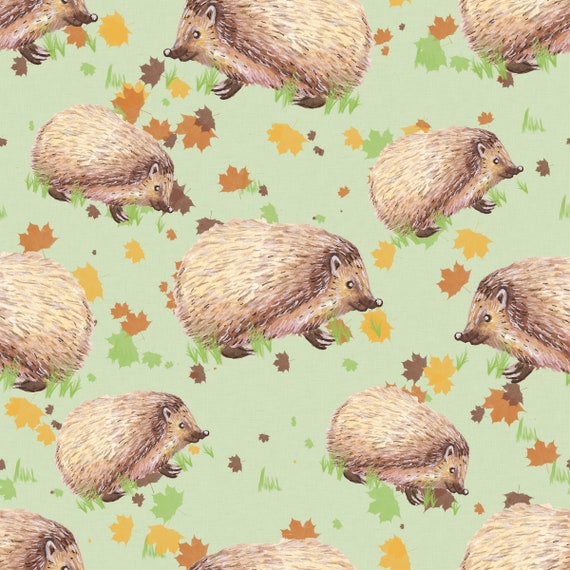The image is a detailed repeating pattern featuring illustrations of a hedgehog. Each hedgehog illustration shows a light brown animal with fur-like spines, a round nose, and small clawed feet, often depicted with a happy face. The hedgehogs are uniformly side-facing and vary in size and orientation, with some facing left and others facing right. The background of the image is a light, mint green, over which scattered colorful leaves - including shades of red, green, yellow, orange, and brown - are placed to evoke the feel of fall foliage. The overall visual motif is simple and charming, making it versatile for various uses such as wallpaper for a child's bedroom, wrapping paper, or scrapbook paper, with a whimsical and country-style aesthetic.